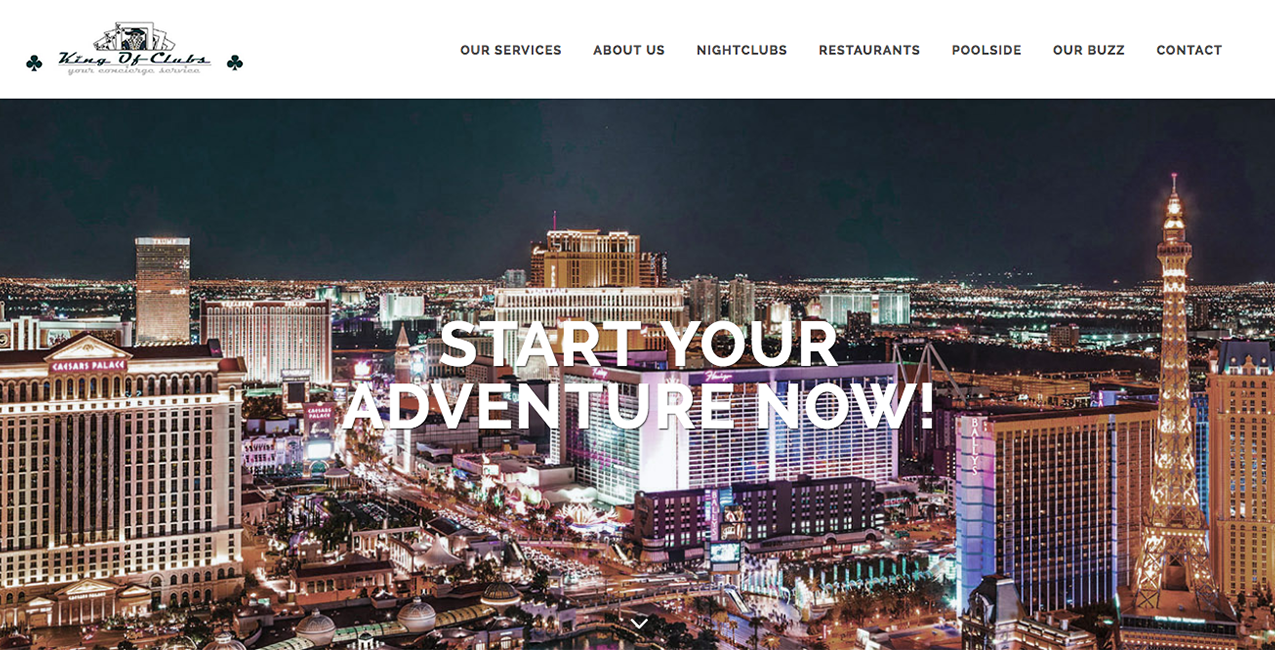A vibrant aerial screenshot of Las Vegas features the bustling cityscape with iconic landmarks highlighted. Dominating the top of the image, an advertisement for the "King of Clubs" showcases two nightclubs on either side of the King of Clubs, surrounded by protruding club symbols. The advertisement includes tabs for "Our Services," "About Us," "Nightclubs," "Restaurants," "Poolside," "Our Buzz," and "Contact," inviting viewers to start their adventure now.

In the heart of the scene, notable landmarks such as Caesar's Palace and the Paris Las Vegas Hotel, famed for their exquisite chocolate martinis, stand out. Adjacent to them, the grandeur of the Bellagio, the luxurious Arras, and the Flamingo are discernible. The city’s heavy traffic is evident, adding to the bustling ambiance. The picture also captures the tram track weaving through the city and new construction near the Flamingo, indicating constant growth. Despite some text overlay about beginning an adventure, the Wynn Hotel can be spotted in the distance. This detailed and dynamic snapshot encapsulates the excitement and continuous evolution of Las Vegas.